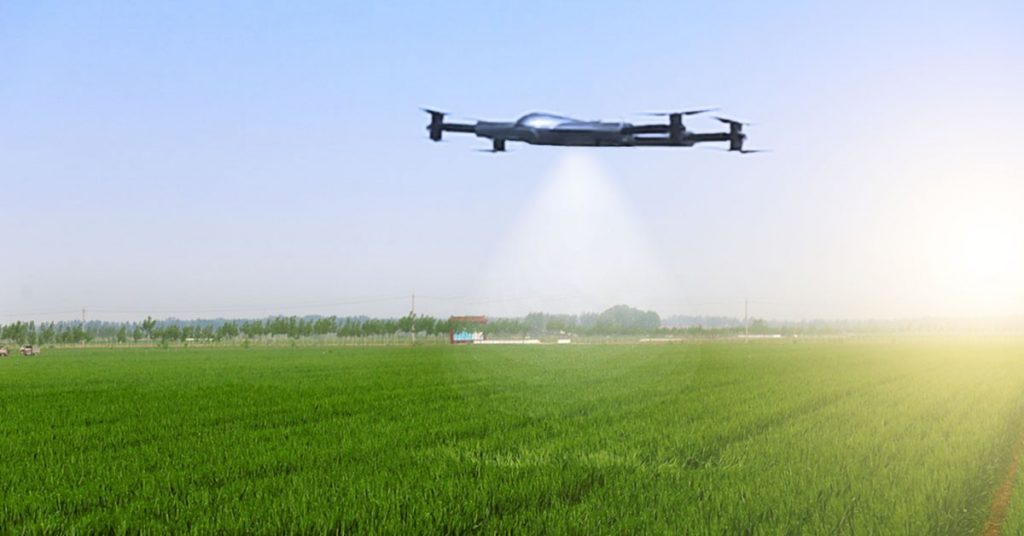In this color photograph taken outdoors during the daytime, we see a detailed scene of a farmer’s field set against a light blue sky that transitions into a foggy or smoggy gray hue towards the horizon. The bottom portion of the image showcases dark green crops stretching across the field. Midway through the picture is a row of tall trees running horizontally from left to right, with a line of storage buildings below them.

Dominating the top center of the photograph is a chrome-colored drone, equipped with propellers on each of its four corners. The drone is slightly to the right of center and is positioned in the sky portion, which makes up about the top two-thirds of the image. It appears to be spraying a white mist down onto the crops in a conical shape, narrower near the drone and expanding wider as it reaches the field below. To the right side of the image, there is a hazy area, either from the mist dispersing or the effect of sun haze, contributing to a realistic, atmospheric depth. The scene is illuminated by the light of a large white and orange sun emerging from the center-right, casting a glow over the misty field. This photograph captures the precise moment of agricultural activity with representational realism.